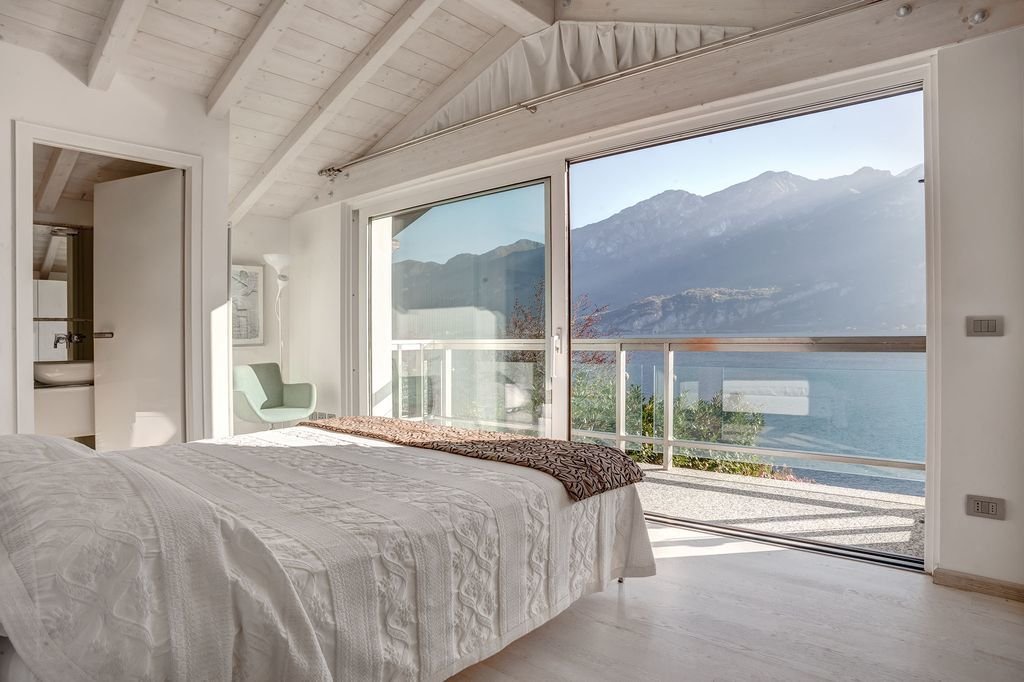This color photograph captures the serene interior of a white wooden cabin, showcasing a room bathed in natural light. Dominating the view in the background, a large window frames a stunning, sunlit landscape featuring a crystal-clear bluish lake bordered by several grayish mountaintops. In the foreground, a bed adorned with a pristine white duvet invites comfort and relaxation. To the left, an open white door reveals a glimpse of an adjoining bathroom, evidenced by a visible mirror. Adjacent to this door, a greenish chair adds a touch of color to the otherwise neutral palette. Completing the scene, a framed picture graces the wall and a white light fixture discreetly illuminates the space. The overall composition exudes tranquility, blending indoor coziness with the breathtaking beauty of the outdoors.